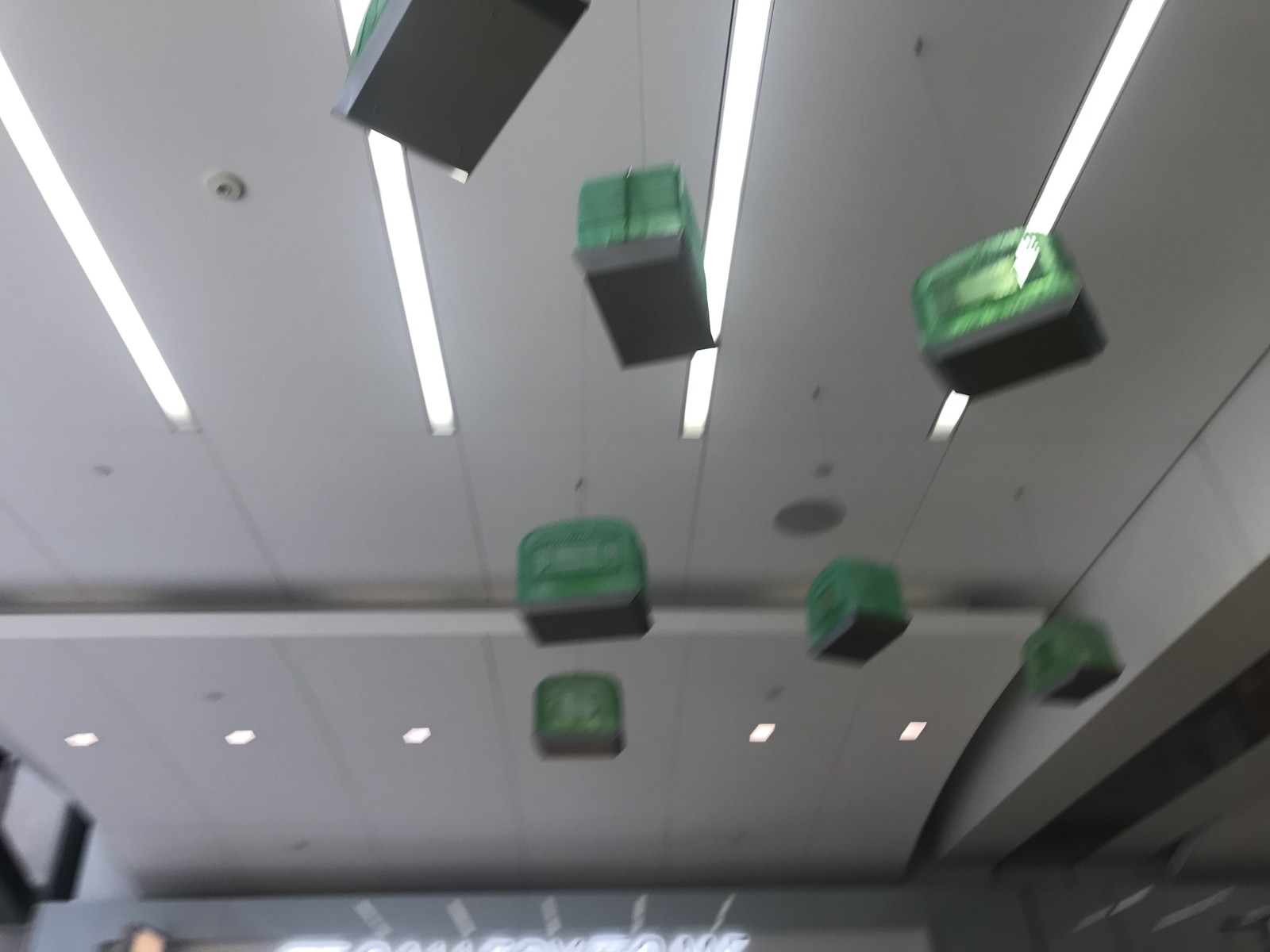This square color photograph, though somewhat blurry, captures what appears to be an artistic installation or display inside a mall or possibly an office-like environment. The focal point consists of seven green rectangular objects, possibly book bags or plastic boxes with black bottoms, hanging from the ceiling by strings. The ceiling, which appears gray and somewhat dingy, features recessed fluorescent and neon lighting as well as commercial sprinklers. Further detail is added with a mounted speaker visible among the ceiling fixtures. Toward the lower part of the frame, a neon sign spans across the background, indicating a storefront or business entrance, though the text on the sign is illegible. The overall impression suggests a creative or whimsical setup within a commercial indoor space.